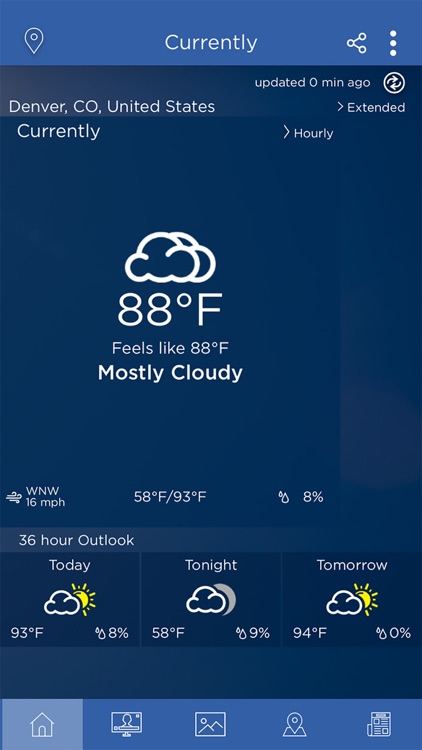This screenshot image predominantly features a blue square. At the top, a lighter blue banner spans the width of the screen. On the upper left corner of the banner, there is a navigation symbol. Centrally positioned within the banner, the text reads "Currently." On the upper right corner, there's an icon symbol followed by a vertical ellipsis (three dots arranged vertically).

The screen displays a weather update. Just below the banner, a message states that the information was updated "0 minutes ago," and beneath this, it says "Extended." Scrolling further down reveals the location: "Denver, Colorado, United States - Currently." 

To the right, there is a section labeled "Hourly" accompanied by a right-pointing arrow.

In the middle section of the screenshot, it shows the current temperature as "88°F" with a statement below it reading "Feels like 88°F," and a description that reads "Mostly Cloudy." 

Continuing to scroll down, the screen indicates wind conditions as "WNW 16 mph." It also notes the day's temperature range: a low of "58°F" and a high of "93°F."

Finally, further detail shows a percentage reading "8%."